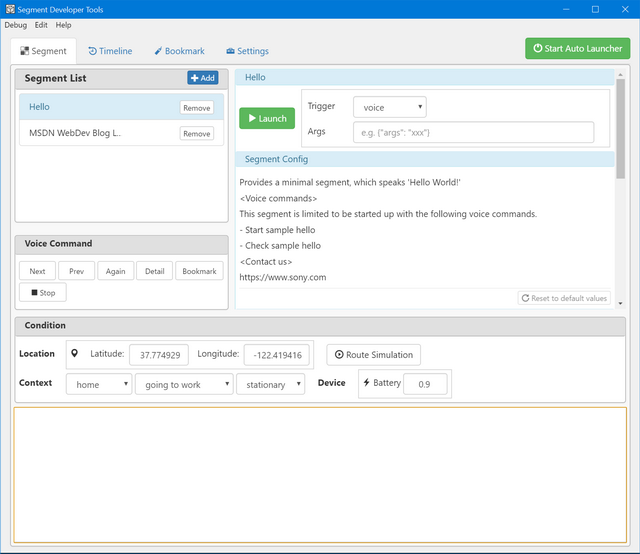The image is a screen capture of a web application featuring an open window titled "Segment Developer Tools." The interface comprises several distinct segments and tabs. At the very top of the window, there are three primary tabs labeled "Debug," "Edit," and "Help." Beneath this, a secondary row features four additional tabs: "Segment," "Timeline," "Bookmark," and "Settings." Notably, the "Segment" tab is highlighted and open.

In the main field of the interface, there is a pane on the left titled "Segment List," accompanied by an "Add" button on its right. Further down, there is a segment displaying the text "Hello," with a "Remove" button adjacent to it. Below that, in capital letters, it reads "NSDN WEB DEV BLOG," also with a "Remove" button to its right. Lower still, there is a small rectangular section labeled "Voice Command," featuring several buttons: "Next," "Preview," "Again," "Detail," "Bookmark," and "Stop."

On the right side of the interface, there is a message window with the text "Hello." Directly below this is a green "Launch" button, alongside options labeled "Trigger" and "ARGS." Further down, a segment titled "Segment Configuration" contains some coding elements. At the bottom of the window, there is an additional section labeled "Condition," featuring another pane with tabs "Longitude," "Latitude," and "Content." Within this section, various options such as "Home," "Going to Work," and "Stationery" are available via dropdown menus. Finally, to the right of these options, a label reads "Device," with a sub-label indicating "Battery."